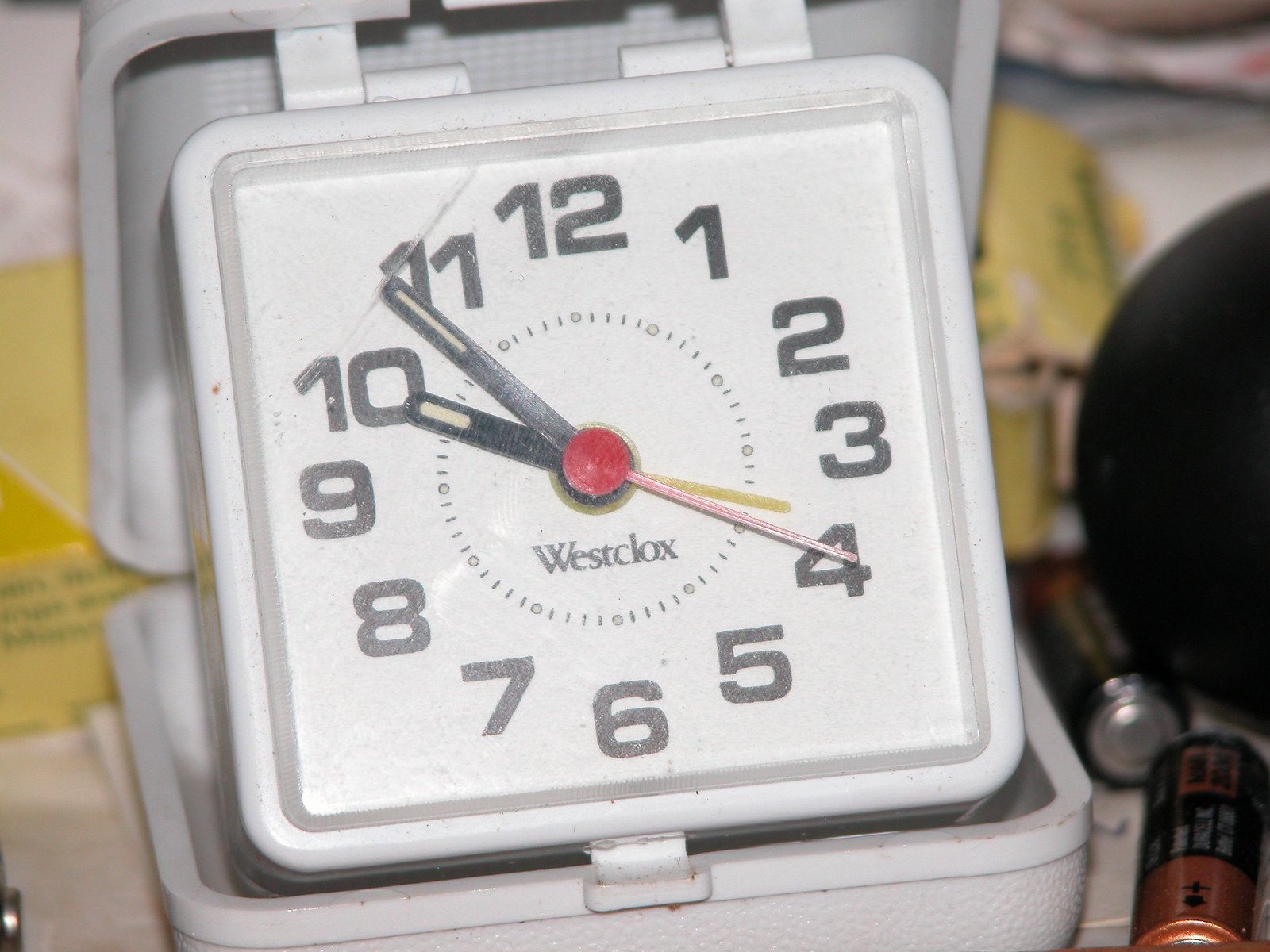This close-up photo features a vintage Westclox travel clock housed in a white or light gray plastic case, possibly foldable. The square clock face is white with black numbers 1 through 12 and minute markers between each number. At the center, there's a red circle. The clock displays the time as 9:53 and 20 seconds, with black hour and minute hands, and a red second hand. Notably, there is also a gold hand, likely for setting the alarm. 

In the background and to the sides of the clock, various items can be seen: several batteries, including one identifiable as a Duracell with a copper top, positioned to the left. The clock face appears slightly aged, with a noticeable crack in the upper left corner. The setting includes a mix of other objects that contribute to the overall scene, such as cartons and a yellowish item behind the clock.